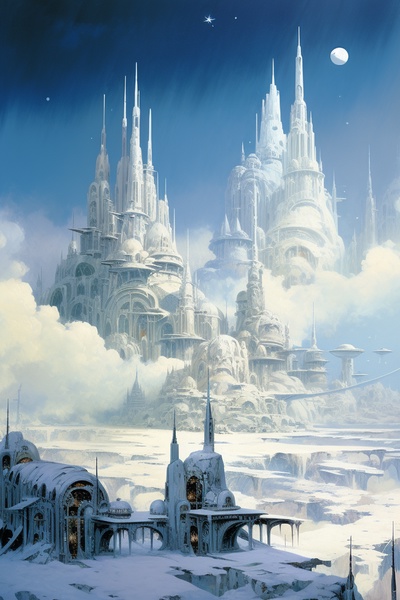The image portrays a fantastical, digitally generated scene featuring majestic, white castles set high in the sky. The castles, intricately detailed with several tall, pointed spires, are enveloped in swirling white clouds, reminiscent of a serene, otherworldly kingdom. Above, a deep blue sky transitions into darker hues, speckled with shimmering stars and a luminous moon. The grandeur of these sky castles is complemented by a smaller, similarly designed building in the foreground, situated on a snow-covered, rocky surface. This smaller structure is connected to the main castles by a snowy, rocky pathway, suggestive of an ethereal bridge to a magical realm. The entire scene communicates a sense of otherworldly awe and fantasy, emphasizing the castles' ethereal and other-dimensional nature.